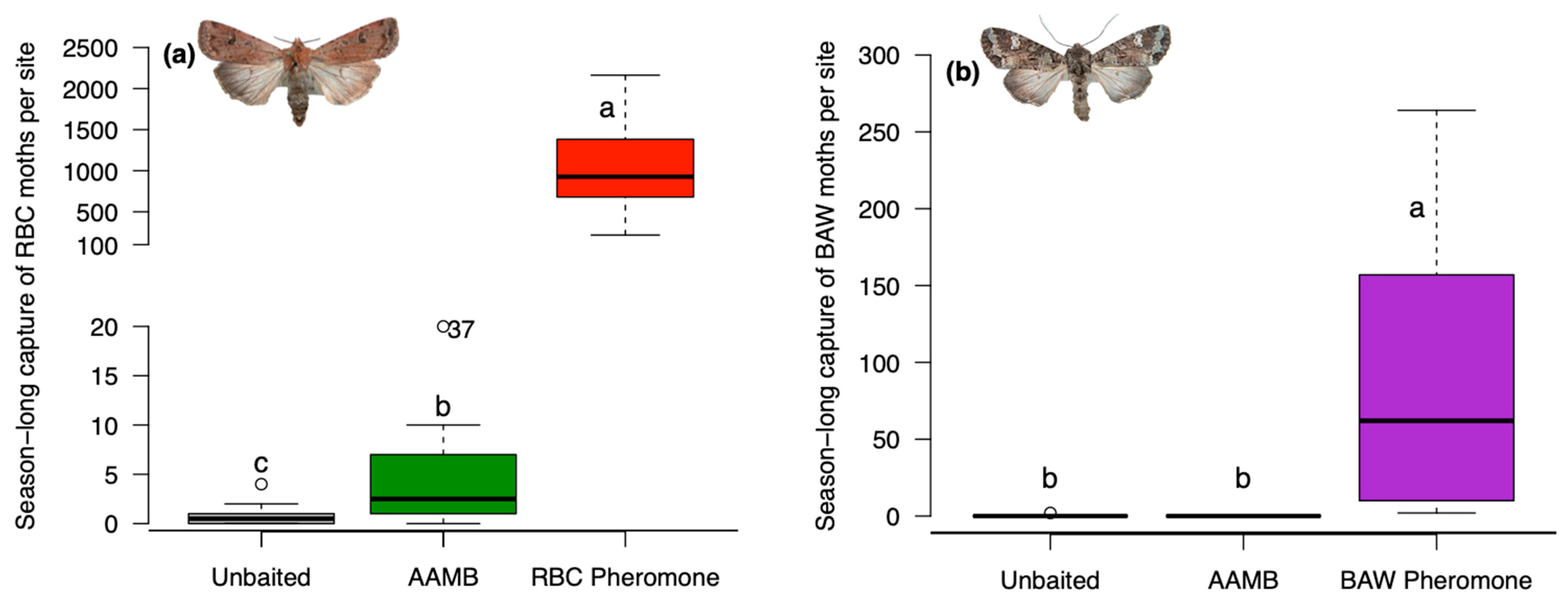The image features two detailed bar charts depicting the season-long capture of two different species of moths per site. The first chart, titled "Season-long Capture of RBC Moths per Site," includes a picture of an RBC moth at the top. The vertical Y-axis, which is segmented from 0 to 2500, quantifies the number of captures. Along the horizontal X-axis, there are three categories: 'Unbaited', 'AAMB', and 'RBC Pheromone'. The 'Unbaited' category shows a tiny black line close to zero, indicating minimal capture. The 'AAMB' category has a green bar reaching approximately 7, and the 'RBC Pheromone' category displays a prominent red bar soaring to around 1000 captures.

The second chart, entitled "Season-long Capture of BAW Moths per Site," features a BAW moth image at the top. This chart also has a similar layout with the Y-axis ranging from 0 to 300 and the same three categories along the X-axis: 'Unbaited', 'AAMB', and 'BAW Pheromone'. The 'Unbaited' section shows minimal capture. The 'AAMB' section displays a green bar, and the 'BAW Pheromone' section is highlighted with a purple bar that peaks close to 300 captures.

Both charts appear to be part of a scientific study comparing moth capture efficacy using different baiting techniques, with noticeable differences highlighted by varying bar colors and heights to represent the capture effectiveness for each type of moth and baiting method.